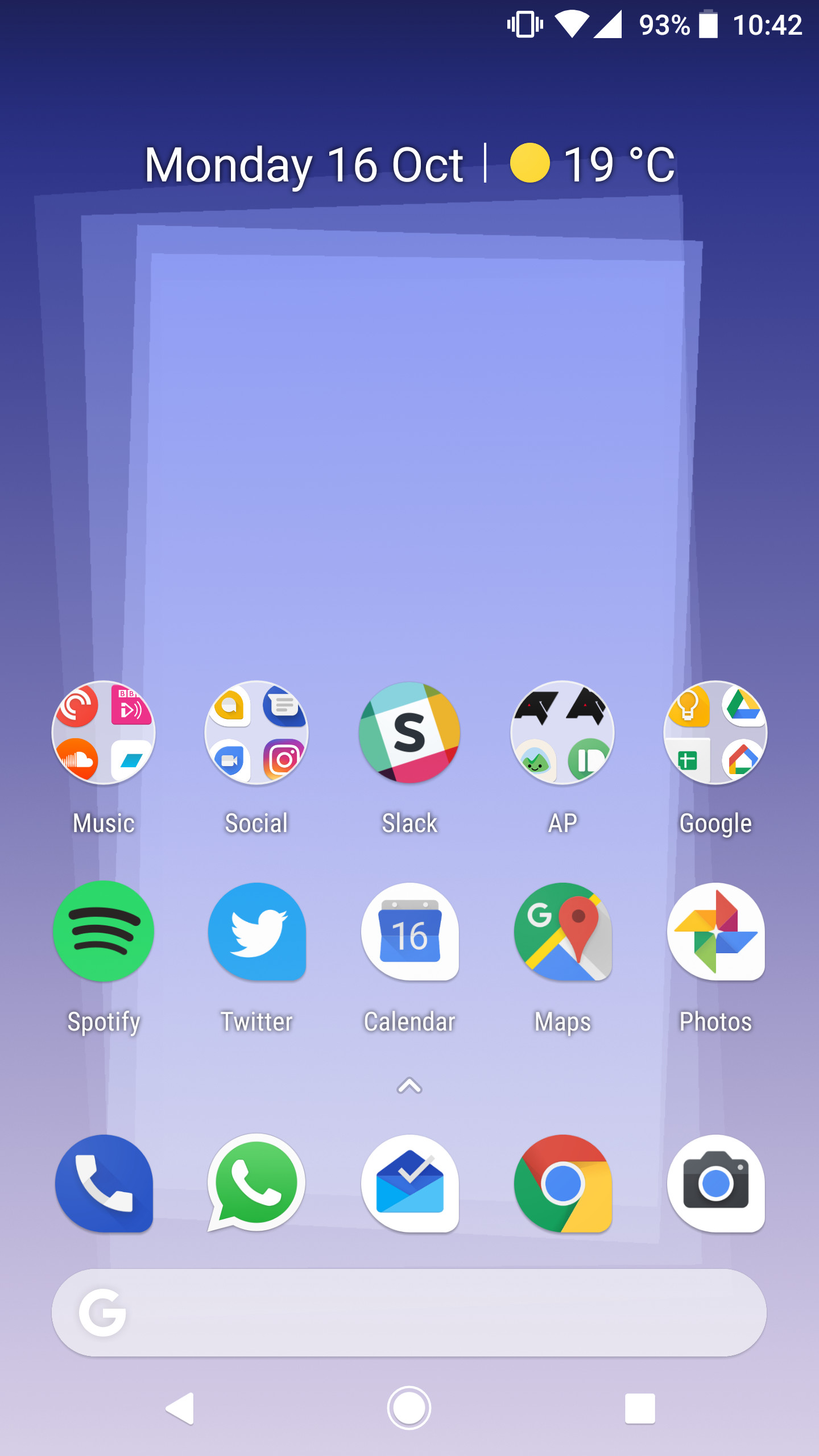This image is a screenshot of a cell phone's home screen, showcasing its wallpaper and various apps. The top right-hand corner displays the time as 10:42 and the battery level at 93%, along with icons indicating cell phone reception and Wi-Fi connectivity. Below this, in white font, it reads "Monday, 16 October OCT," followed by a vertical line and a yellow sun icon indicating a temperature of 19°C.

The screen is organized into three rows of apps, with each row containing five apps. The top row includes a music app, a social media app, Slack, AP, and Google. The middle row features Spotify, Twitter, Calendar, Maps, and Photos. The bottom row consists of the Phone app, Messaging app, Email, Google Chrome, and the Camera app.